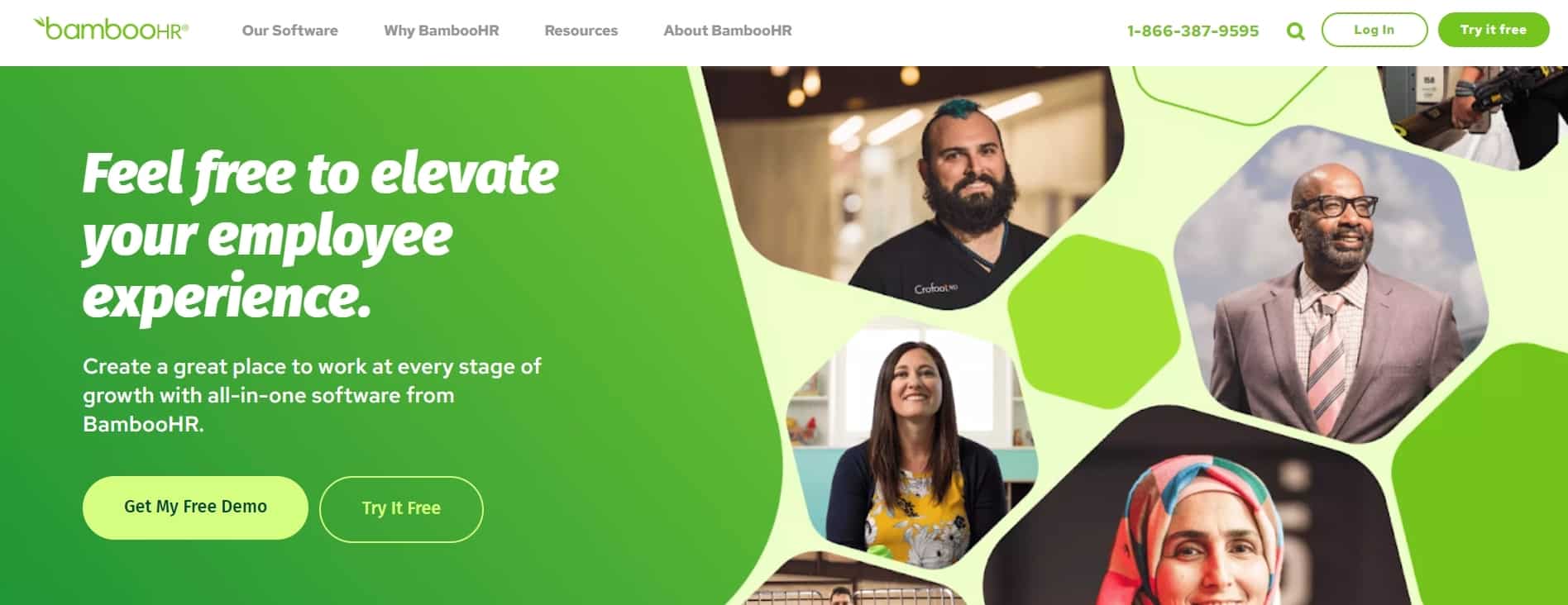This screenshot captures the homepage of Bamboo HR, featuring a clean and organized layout with distinct sections and visual elements. At the top, there is a white banner with the Bamboo HR logo on the upper left corner in green text. Adjacent to the logo are navigation options including "Our Software," "Why Bamboo HR?" and "Resources about HR." On the upper right, a green phone number (1-866-387-9595) is displayed, followed by a magnifying glass icon (presumably for search), a login button, and a prominent green "Try It Free" button in white text.

The main section of the page is divided into two contrasting backgrounds: green on the left and yellow with irregular green spots on the right. The left side features a bold headline in white text: "Feel Free to Elevate Your Employee Experience." Below this is a subheading that says, "Create a great place to work at every stage of growth with all-in-one software from Bamboo HR." Two call-to-action buttons, "Get My Free Demo" and "Try It Free," are positioned beneath the text.

On the right side of the page, the section is filled with irregularly shaped spaces containing photographs of diverse individuals. Among them is a man with dark hair and a beard, smiling directly at the camera; a woman with shoulder-length dark brown hair, slightly tilting her head up and smiling, dressed in a yellow flowered dress and black cardigan; a woman wearing a multi-colored hijab (pink, blue, and pale green), also smiling and facing forward; and a dark-skinned man with glasses, a beard, and a bald head, dressed in a gray suit, looking towards the right. These images contribute to the inclusive and friendly atmosphere the website aims to convey.